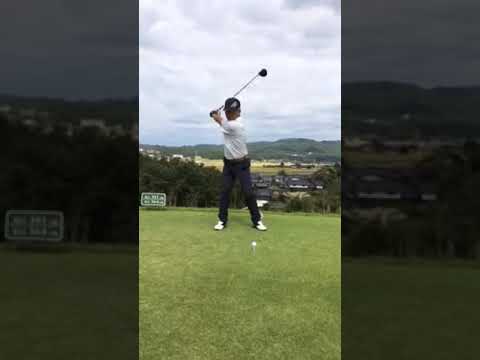In this richly detailed photograph set on a picturesque golf course, a man is poised to swing a wood club high above his head, preparing to strike a white golf ball teed up in front of him. He is attired in a white golf shirt, dark blue trousers, white sneakers, and a black cap adorned with a small, indistinguishable white symbol. The scene features a meticulously mowed grassy tee box, with a green sign bearing white numbers to his left. Surrounding him, the course is lush with greenery, bordered by tree lines that flank a gently sloping hill. In the background, several buildings are nestled at the hill’s base, leading up to majestic mountains under a sky dotted with both white and slightly blue-tinged clouds. The predominance of the verdant grass enhances the natural beauty of the golfing landscape.